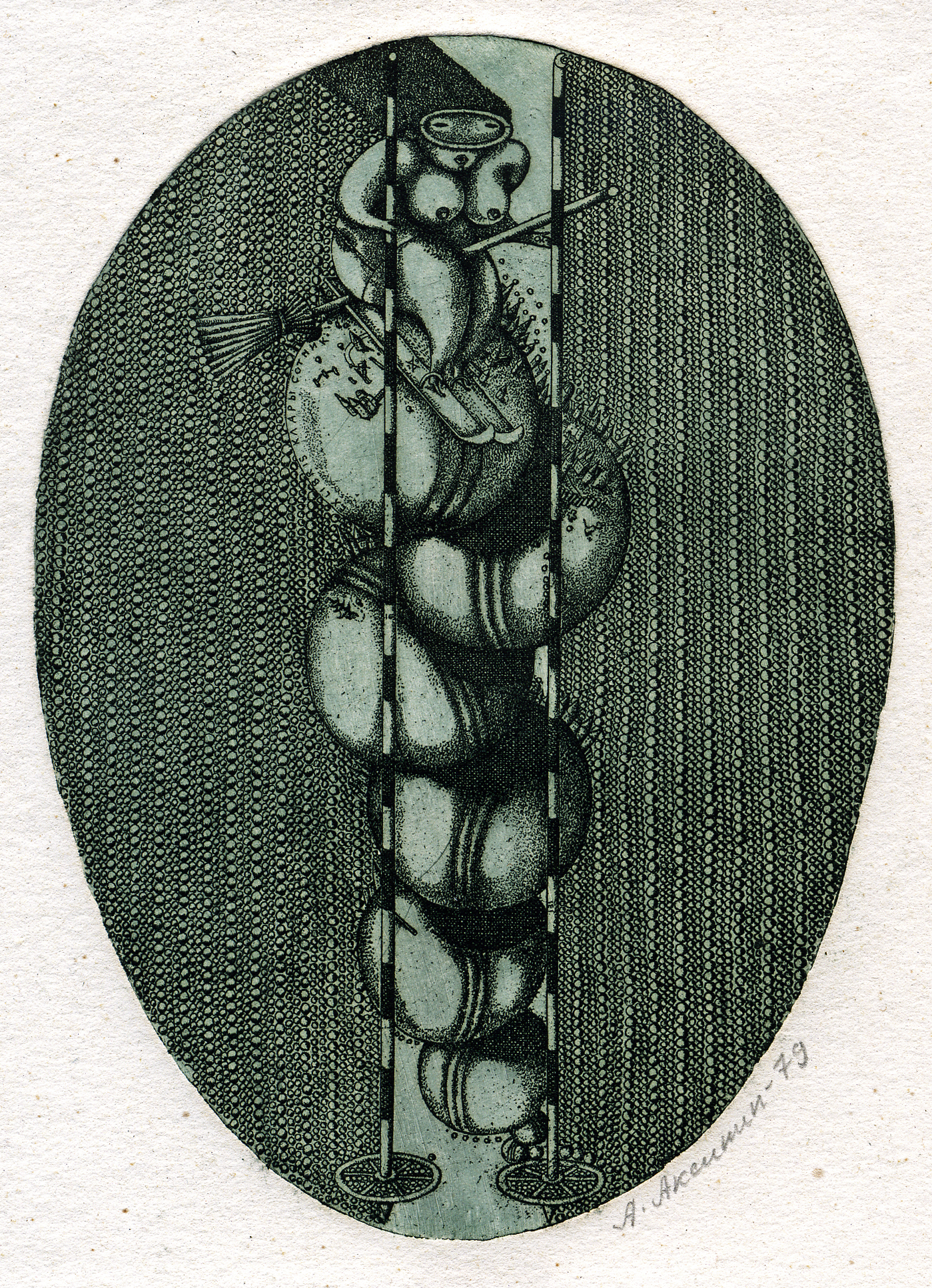The abstract, surrealist artwork features a central gray and green oval against a rectangular, white background with scribbled text that might read "79." Encircling the oval is an array of small, ball-shaped patterns aligned in numerous columns. Dominating the middle of this oval is a striking depiction of a nude woman. Her breasts are visible, and she wears a scuba diving mask. The woman is positioned as though skiing, with skis on her legs and a broomstick between her thighs. This fantastical scene includes six vertically stacked balls, resembling golf balls, beneath her. She is flanked by two very long, vertically striped poles that extend from the top to the bottom of the oval, adding to the artwork's surreal and distinctive composition.